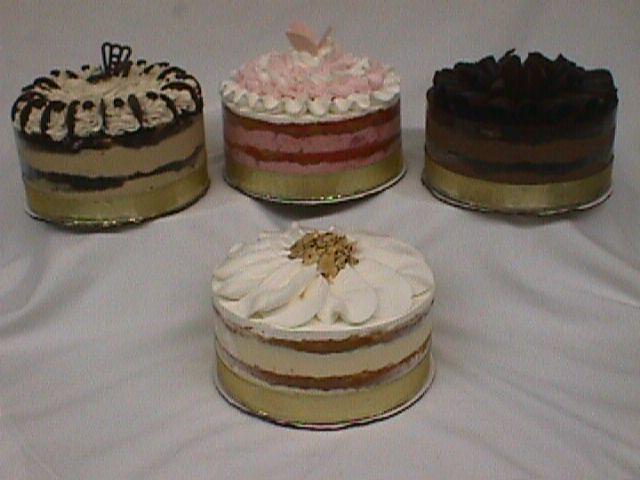The photograph captures four elaborately decorated round cakes displayed on a surface draped with a wrinkled white cloth that adds texture and dimension to the background. The setup resembles a tiered shelf with three cakes elevated in the back row and one cake positioned in the foreground. Each cake is perched on a gold stand, adding a touch of elegance to the presentation. 

The cakes, each with four to five layers, exhibit a variety of colors and textures. The cake in the foreground features a white icing top with small nuts in the center, atop layers of medium tan and brown stripes. In the back row, the cake to the left is adorned with chocolate frosting and dark chocolate pieces that resemble Oreo cookies. The middle cake stands out with its vibrant pink and red striped layers, topped with pink and white icing. The far-right cake showcases dark chocolate icing with lighter chocolate stripes, also finishing with a gold bottom layer.

This detailed arrangement not only emphasizes the intricate designs of each cake but also highlights the textured, non-uniform background that adds depth to the presentation.